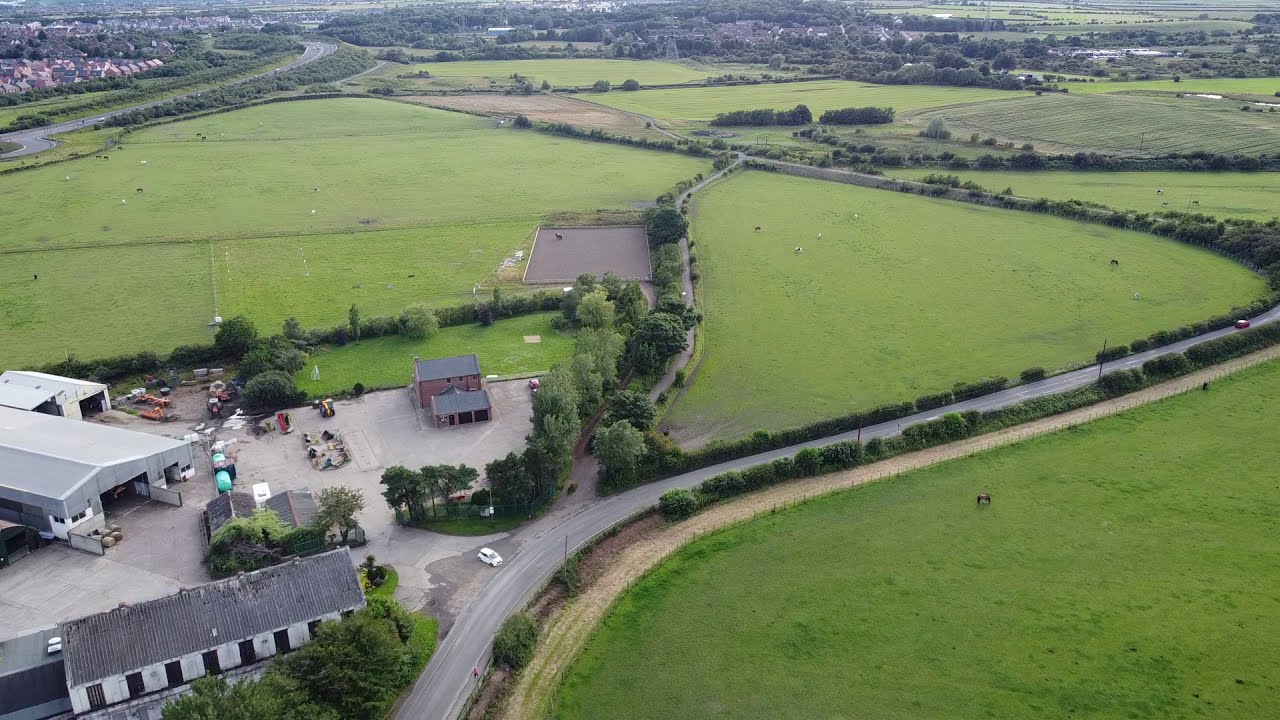This detailed aerial photograph captures a sprawling rural landscape characterized by expansive grassy fields and scattered clusters of buildings. On the lower left side, a sizable compound features multiple structures with gray and metal roofs. The central focus is a large, industrial-looking warehouse with its door ajar, adjacent to a smaller building marked by numerous windows and doors. Surrounding these buildings is an extensive concrete slab or parking lot, suggesting a mix of residential and business use. Nearby, colorful farm equipment, orange tractors, and blue tanks dot the area, indicating agricultural activities.

A long, winding road traverses the scene from left to right, lined with smaller trees and bushes, eventually opening into broader meadows and pastures. These green pastures, dotted with animals that might be horses or cows, extend across the landscape, adding to the bucolic charm. Dominating the center of the image is a large square pen or corral, potentially for horses, characterized by an unusual grayish floor, which could be dirt or clay.

In the distance, a small town peeks through a canopy of taller trees, adding depth to the rural vista. The combination of open fields, varied buildings, and gently curving roads conveys a serene yet industrious countryside scene.